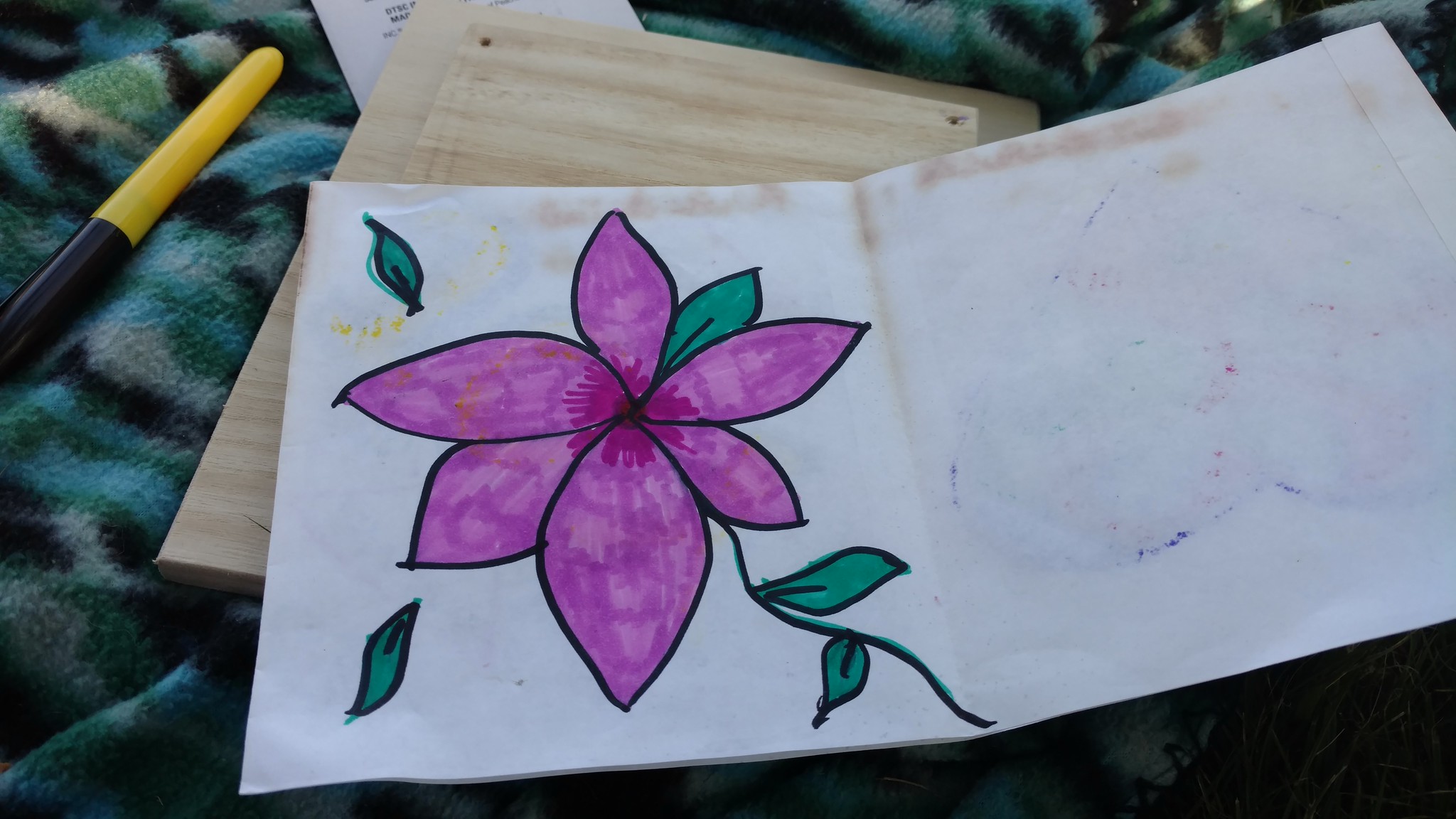A beautifully illustrated watercolor painting graces the center of a pristine white sheet of paper, showcasing a vibrant flower with six deep violet petals. Each petal radiates saturated color, drawing the eye toward the lush green stem adorned with three verdant leaves. Two additional deep green leaves lie to the left, seemingly separated from the main floral figure. The paper rests atop a sturdy page board, which in turn is laid out on a luxuriant deep green blanket, creating a striking contrast that adds depth to the composition.